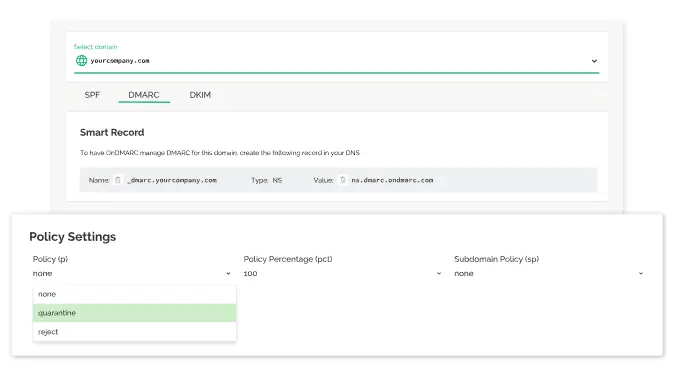A screenshot of a web page for ONDMARC, featuring a predominantly white, green, and black color scheme. At the top of the page, there is a header with the text "Select Location" in green font alongside a green globe icon and the text "yourcompany.com" in black. To the right of this header, there is a drop-down menu and a prominent green navigation bar.

Below the header, a series of tabs are visible, with 'FISPF' and 'DMARC' in gray and underlined in green, and 'DKIM' in black, indicating the user's current section. The page content focuses on managing DMARC records for a client. Instructions are provided for creating a DNS record with the following details: Name - DMARC.yourcompany.com, Type - NS, and appropriate values.

Further down, there is a larger, rectangular box titled "Policy Settings" in black text. The policy setting options are displayed, with 'None,' 'Quarantine' highlighted in light green, and 'Reject.' Additionally, the policy enforcement percentage is set at 100%, and the subdomain policy is marked as 'None.' The overall presentation is clean and functional, aimed at guiding users through configuring their DMARC settings.